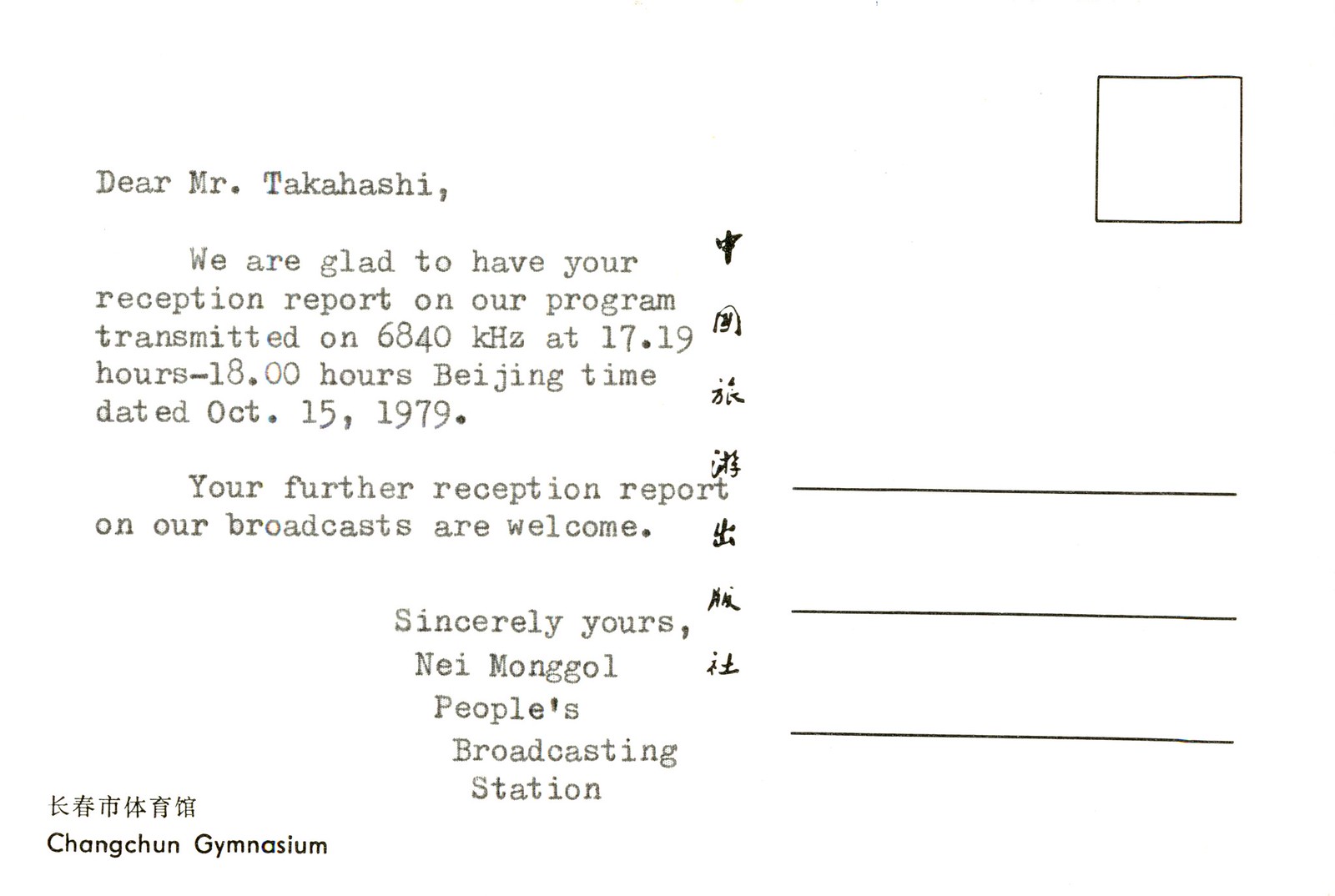The back of the postcard features a typewritten note on the left side that reads: "Dear Mr. Takahashi, we are glad to have your reception report on our program transmitted on 6840 kHz at 17.19 hours to 18.00 hours Beijing time dated October 15th, 1979. Your further reception report on our broadcasts are welcome. Sincerely yours, Nei Monggol People's Broadcasting Station." Below this note, printed on the postcard, it says, "Changchun Gymnasium," accompanied by a string of eight Chinese characters. The right side of the postcard is blank, featuring a square in the top right corner intended for a stamp, and below it are three horizontal lines designated for address information. The overall surface of the postcard is white.